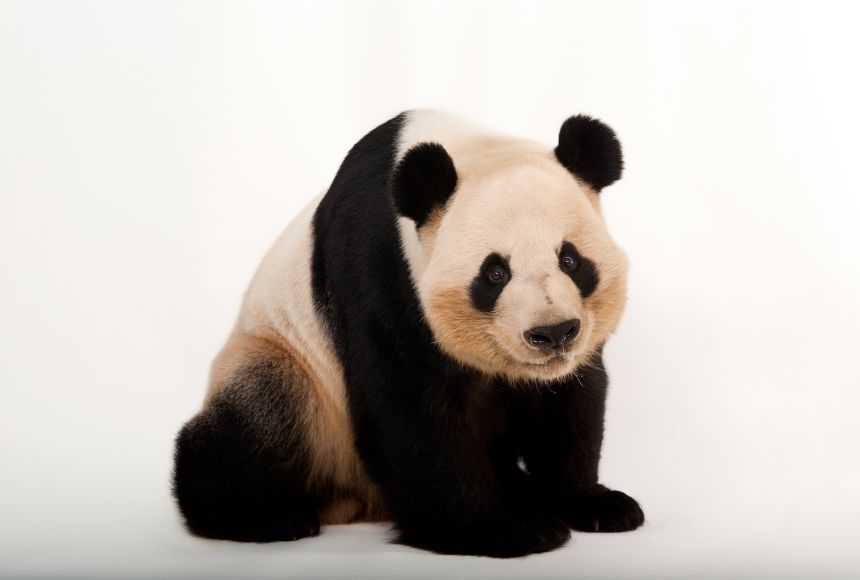This is a horizontal, color, rectangular image featuring a live adult panda bear seated and facing the camera, captured as if in a studio or created using AI. The background is entirely white with a light gray floor. The panda, with an endearing and neutral expression, exhibits the classic black-and-white coloration typical to its species, along with some unique features. Its broad white face has tinges of beige and cream, while the area around its eyes, ears, and large nose is entirely black. The fur on its shoulders and back displays a mixture of black, white, and some brown, especially along the haunches. The panda's front and back paws are black, though slightly blurred. The stark white background emphasizes the details of the panda, making it look like it’s posing for the photo.